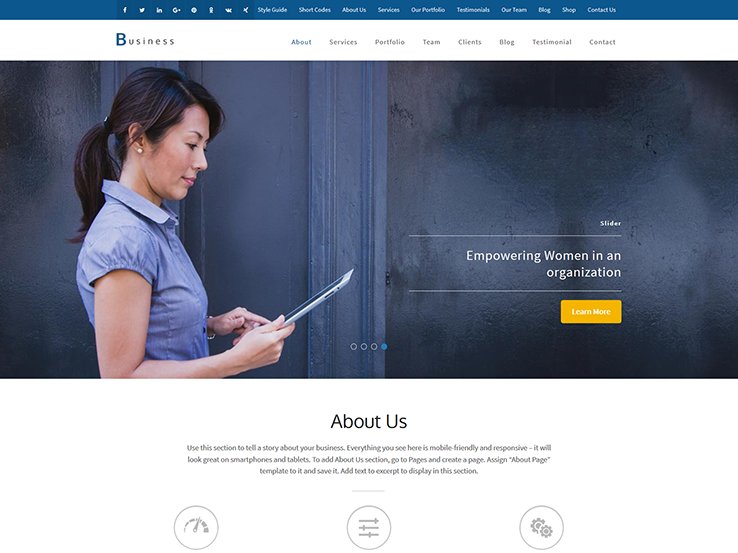A screenshot of a website is shown with a blue banner stretching across the top. This banner features navigation links labeled "Style Guide," "Short Codes," "About Us," "Services," "Our Portfolio," "Testimonials," "Our Team," "Blog," "Share," and "Contacts." The "Style Guide" link appears to be selected.

Below this is a white section prominently displaying the word "Business" with a large blue 'B,' accompanied by smaller gray text. This area offers links named "About," "Services," "Portfolio," "Clients," "Blog," "Testimonials," and "Content."

Positioned centrally is an image of a woman with her hair styled in a tight ponytail, looking intently at an iPad. Her focus is directed towards the device, and she stands before what appears to be a chalkboard set against a very faded blue wall. She is dressed in a blue or violet top. Overlaying this image is a text box that reads "Slides: Empowering Women in an Organization," accompanied by a clickable yellow button labeled "Learn More."

Towards the bottom of the webpage is an "About Us" section, instructing users to use this part of the site to share the story of their business. It affirms that the entire website is mobile-friendly and responsive, ensuring a visually appealing display on both smartphones and tablets. Additional directions are provided for adding an "About Us" section by creating a page, assigning it the "About Page" template, and saving it, with text excerpts displayed in this area. There is also a mention of downloadable content available on the site.